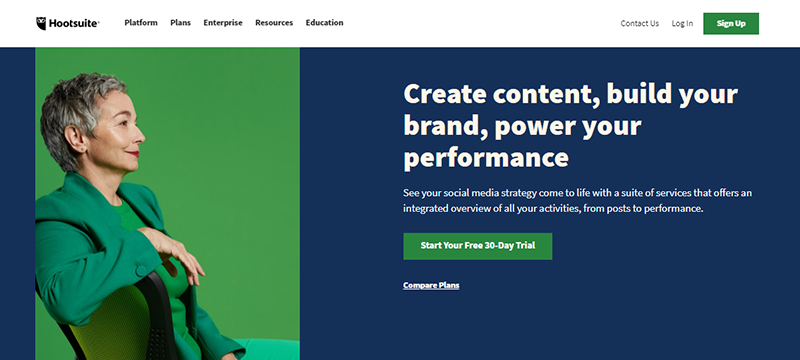The Hootsuite website is prominently displayed, with the company name in black font at the top left corner. Accompanied by an owl icon peeking from the side, this logo is a distinctive visual marker. To the right, there are five navigational categories: Platform, Plans, Enterprise, Resources, and Education, all in black font. Located at the far right, three options are visible: Contact Us, Login, and Sign Up. The Sign-Up option stands out in a green box with white font, while the other two are set in black font on a white background.

Beneath this header, a dark blue box spans the width of the page. On the left side of this section, a woman in a completely green outfit sits on a matching green chair against a green background, creating a cohesive and striking image. To the right, a bold white font delivers the message: "Create Content, Build Your Brand, Power Your Performance." Below this bold statement, a smaller white font elaborates: "See your social media strategy come to life with a suite of services that offers an integrated view of all your activities from post to performance." Directly beneath this, a green box with white font invites users to "Start Your Free 30-Day Trial." Finally, an underlined, small bold white font points to the option to "Compare Plans."